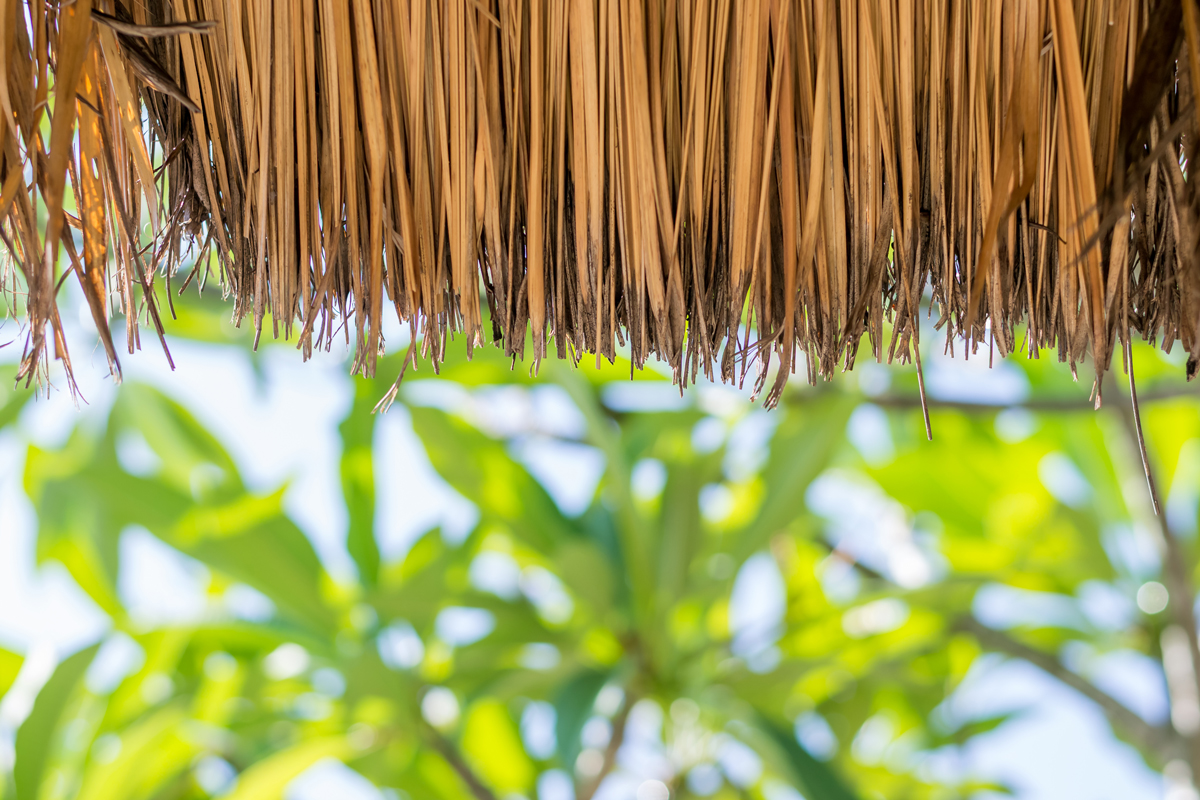This photograph, captured in landscape orientation, features a detailed scene shot from beneath a structure with a palm frond thatched roof, likely resembling a tiki bar or tropical hut. Hanging from the unseen roof are densely packed, dry, needle-like palm fronds that are light brown to orangish in color. These fronds are nearly uniform in length, forming a boundary-like shape at the top of the image. The backdrop is slightly blurred, revealing a combination of green leaves and a clear, bright sky with shades of white and light blue. This contrast in focus emphasizes the tropical setting and the structure's rustic roofing material.